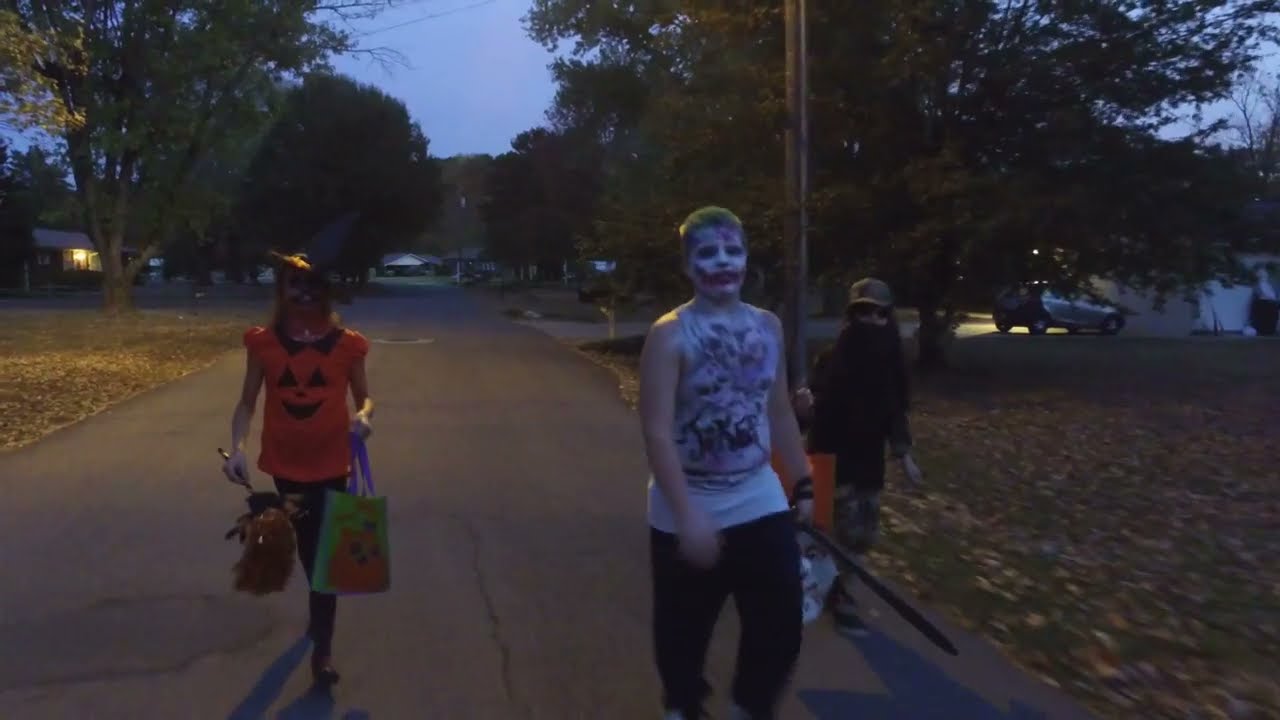The image captures a nighttime Halloween scene on a residential street in a small town, with houses and trees lining the road. There is a light pole behind the group, and a vehicle is parked in the driveway of one of the houses in the background. Three kids are trick-or-treating, walking towards the camera. On the left, a child is dressed as a jack-o'-lantern, wearing an orange shirt with jack-o'-lantern features, black pants, and a witch's hat. They are holding a green trick-or-treat bag with purple handles in their left hand and something indistinguishable in their right. The middle child appears to be dressed as the Joker from Batman, with green hair, white face paint accented with red around the mouth, a sleeveless white shirt, and black pants; they are carrying a bag in their left hand. The third child, slightly behind the others on the right, is wearing fatigue-colored pants, a black shirt, a black face mask resembling a ninja, and a cap, also carrying an orange bag. The pavement shows signs of weathering and cracks, while the lawns are strewn with fallen leaves, emphasizing the autumn season.